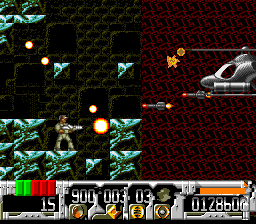This detailed image captures the essence of a retro, side-scrolling, pixelated video game, reminiscent of classic titles on the Super Nintendo or Sega consoles, similar to Contra. On the left side of the screen stands the player character, a soldier garbed in green military gear and wielding a silver rifle, shooting orange fireballs. He is positioned on green-blue blocks, backed by a diamond-patterned wall. The soldier is engaged in combat with a silver helicopter stationed on the right side, which counters with grey missiles. The helicopter is set against a red and black patterned background. At the bottom of the screen, a silver bar displays various game parameters: two green bars and three red bars on the far left, followed by the numbers 15, 900, 003, and 03 alongside indicators such as symbols, an orange-centered diamond, eyeballs, a grey smear, and a score of 012860 topped with an orange bar. This interface likely represents the player's score, life, ammunition, and other vital statistics, encapsulating the nostalgic feel of early video games.